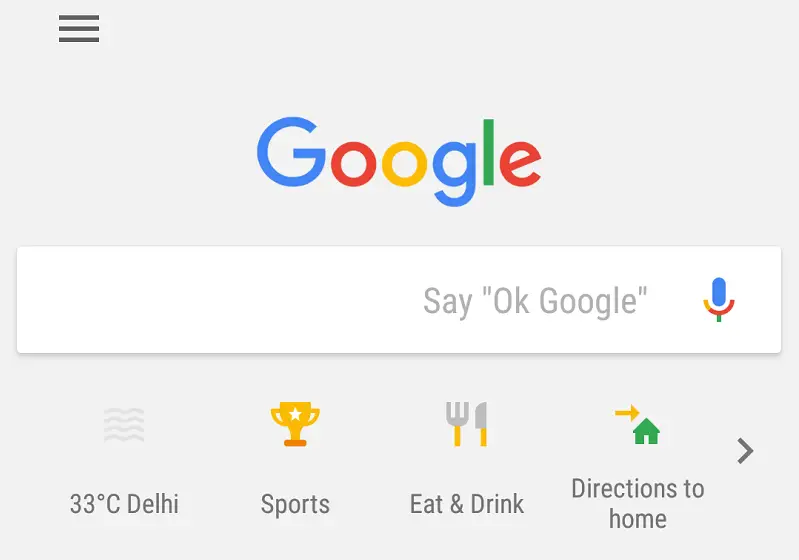A screen capture of a Google search interface showcases the familiar Google logo in its signature multicolored letters prominently at the top. Positioned below the logo is the search bar, featuring a small microphone icon on the right side with the instruction "Say 'OK Google'" next to it, indicating how to activate the voice command feature. Below the search bar, there is a snippet displaying the current temperature in Delhi, reading "33 degrees Celsius." The screen also includes four distinct icons representing different Google services: a weather app, a sports update feature, an "Eat and Drink" recommendation service, and directions to the user's home. This particular layout of the Google search interface could be an older version, a highly-customized setup by the user, or a localized version specific to India that might differ from those available in North America.